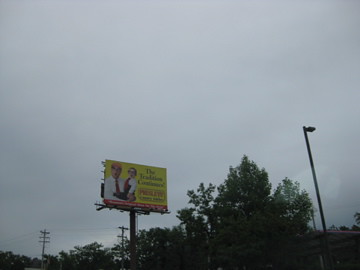The photograph captures a dark, overcast sky suggesting an impending storm, evidenced by the trees swaying in the wind. At the center of the image, there is a yellow billboard located at a distance. The billboard features a man in a white shirt and red tie, wearing a baseball cap and glasses, holding a smaller figure, possibly a child dressed similarly or a ventriloquist dummy, also wearing glasses. The background of the billboard is yellow, with some text in green and red, though the specifics are not legible. Surrounding the billboard are power lines and streetlights, with electricity poles peeking out from the tops of the trees. The entire scene is framed by the brooding, cloudy sky which dominates the upper portion of the photograph.